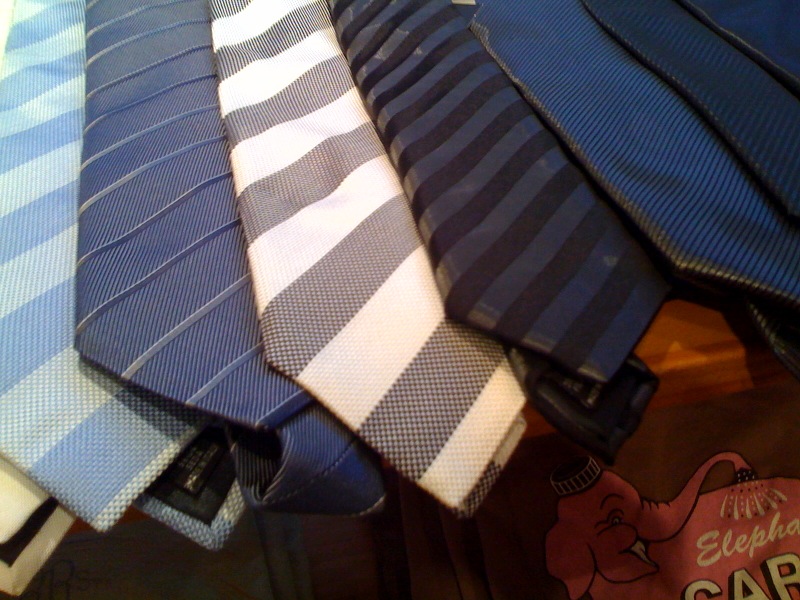The image features the bottom parts of seven neckties laid out on a wooden surface, all aligned with their ends facing the viewer. Each tie showcases a unique diagonal stripe pattern, predominantly featuring various shades of blue, gray, and black. From left to right, the first tie has light blue and dark blue diagonal stripes, the second displays dark blue and gray stripes, the third is white and gray striped, the fourth exhibits navy blue and black stripes, and the remaining three ties also follow a similar navy blue and black diagonal stripe pattern. Additionally, at the bottom right corner of the wooden surface, there is a picture of a pink elephant wearing a black cap. The image also contains some yellowed text, partially obscured, but discernible words include "elephant" and the letters "A&R".